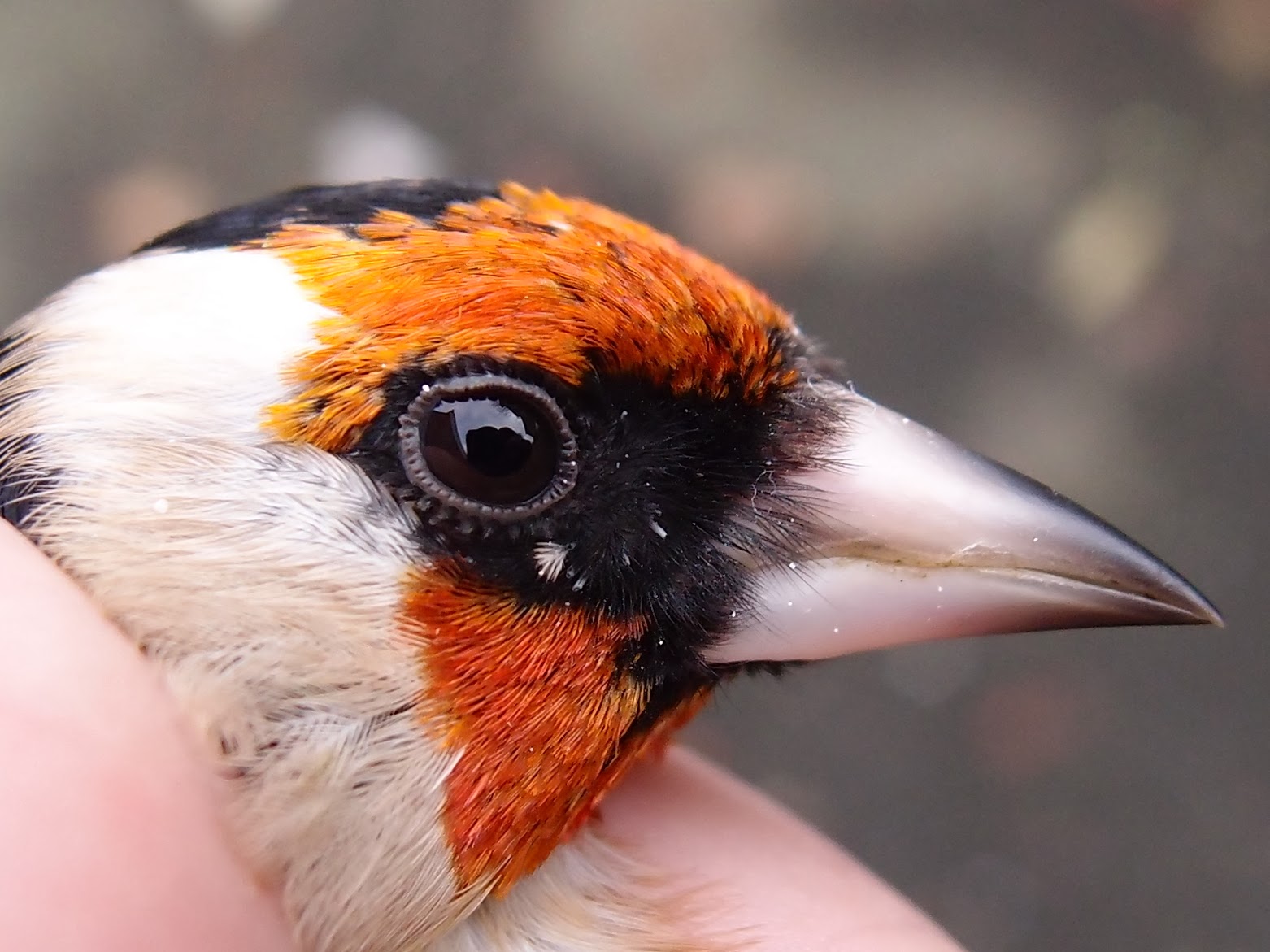This close-up horizontal photograph showcases the striking head of a bird being gently held, with a finger on one side of its neck and a palm on the other. The bird's head features a captivating blend of colors: a vibrant orange crown transitions into a band of black surrounding its liquid black eye, which is wide open and brimming with detail. Below the black band, the orange reappears, framing its long, sharply pointed beak that is primarily light-colored but darkens towards the tip with shades of gray and black. There are white feathers visible near the bird's beak and eye, possibly contaminated with small particles or debris. The intricate texture of the bird's feathers and the fine ridges around its eye are crisply focused, while the background remains a soft, blurred mix of gray, white, and green, drawing full attention to the bird's magnificent and serene profile.